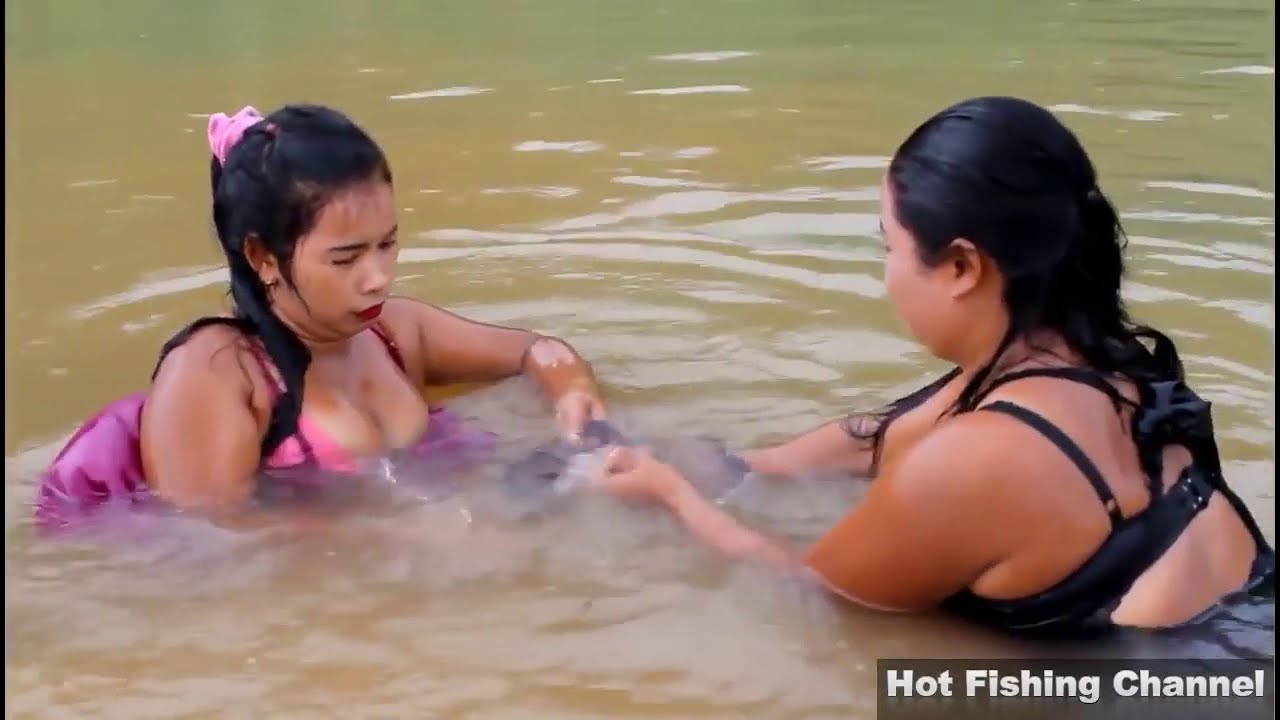In the image, two young women appear to be in their 20s, immersed in a murky river or lake. The woman on the left wears a pink dress that billows around her in the water and has a matching pink hair tie securing her black hair, styled in a ponytail. She also sports red lipstick and has her eyes closed, revealing a neutral expression. Though slightly overweight, she has a graceful presence. The woman on the right, predominantly seen from the side, is dressed in a black swimsuit comprising a bra and possibly a skirt. Her dark, wet hair adds to the vivid scene. The water they are in displays a muddy brown and green hue, adding to the earthy tone of the image. Both women hold unidentified objects in their hands. The scene is captioned with "Hot Fishing Channel" in the bottom right corner, suggesting a casual or playful fishing adventure.